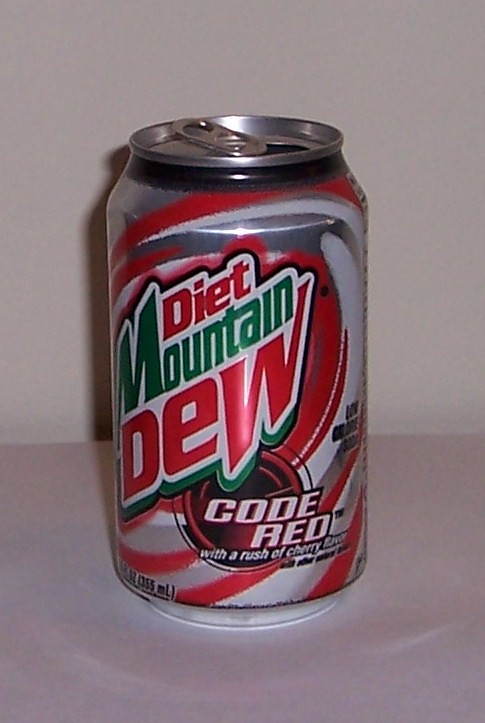The image is a detailed color photograph of a Diet Mountain Dew Code Red can, centered on a white surface with a white background. The can is standard aluminum with a flip-top lid that has been opened, indicated by the dark hole where the tab has been pushed down. The primary design features swirling broad strokes of red and white against the polished silver aluminum background. "Diet" is in red text, "Mountain" in green text, and "Dew" in large, diagonal red letters, consistent with the iconic Mountain Dew script. Near the bottom of the can, within a black circle, is a red logo that reads "Code Red," highlighting the rush of cherry flavor. The vibrant design and bold text create a striking visual impression, emphasizing the soda's distinct branding.